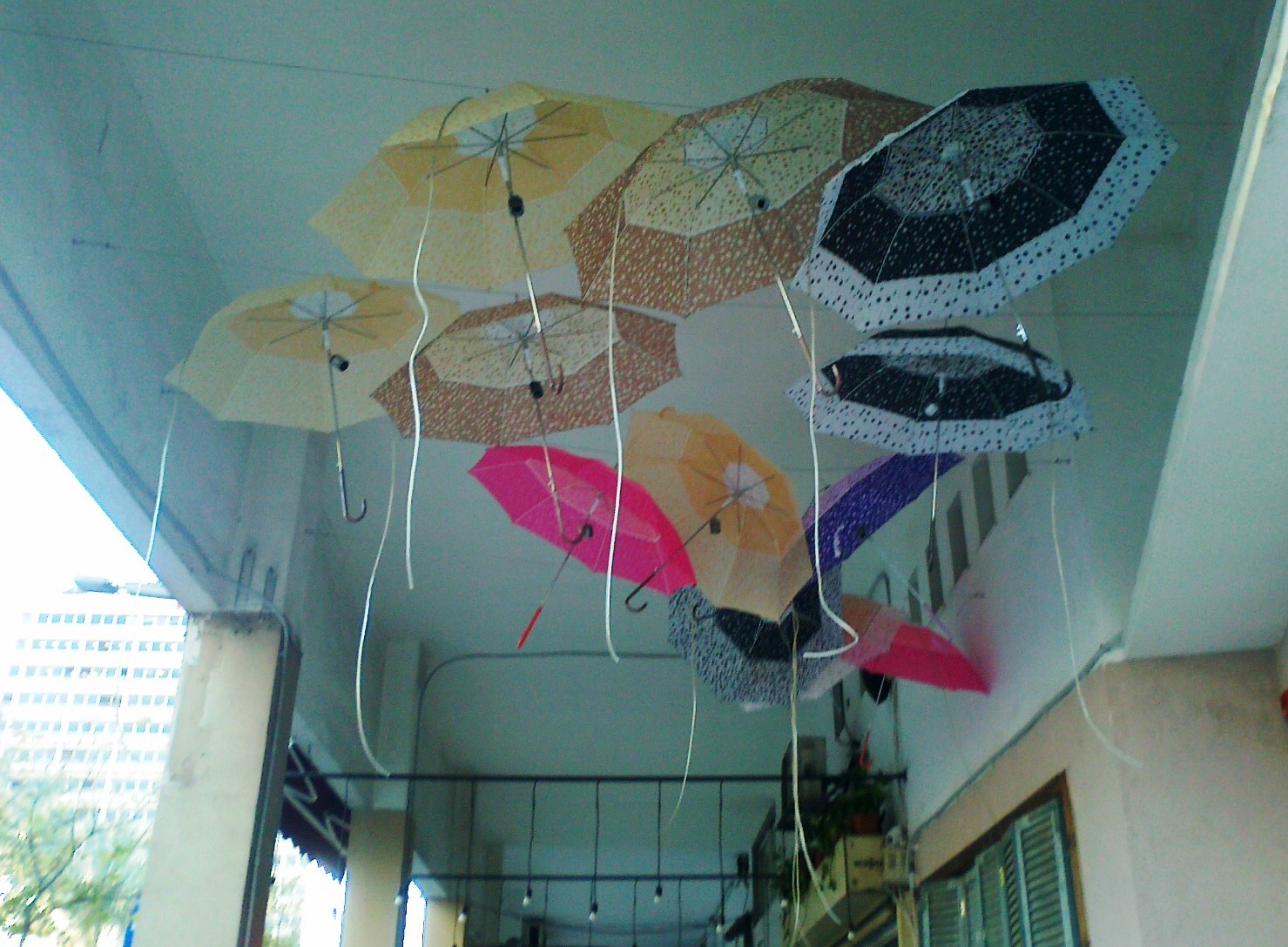In this photograph, we observe a visually striking display of eleven open umbrellas hanging from wires across the ceiling of a covered outdoor area, possibly part of an apartment complex or similar setting. The umbrellas come in a variety of colors: there are three yellow, two brown with speckles, three black and white (some with reversed color patterns), two bright pink, and one purple. The umbrellas are suspended by strings, which hang down from a light green ceiling. The area features elements of beige-colored pillars and cement walls. 

Additionally, the scene includes rows of hanging patio lights, adding to the ambiance. On the left side of the image, beyond the covered space, a high-rise building and a tree with green leaves can be seen, emphasizing the outdoor, yet partially sheltered, nature of the location. The photograph captures a blend of artistic display and functional architectural features set against a backdrop of urban elements.